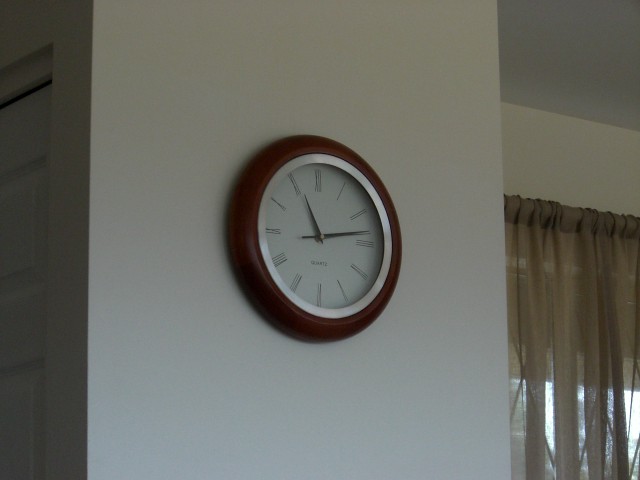A contemporary photograph captures a clock prominently displayed on a narrow hallway wall. The clock features Roman numerals and slender hands, notably lacking a second hand. It is encased in a bezel made of dark-colored wood with a silver inner rim encircling the clock face. To the left side of the image, there is the edge of a doorway visible, suggesting another room around the corner. On the right side, part of the ceiling is visible along with sheer curtains hanging, which are translucent and brown in color, allowing a subtle view of the wall behind them. The combination of the clock's classic design and the modern elements of the space creates an intriguing blend of styles.